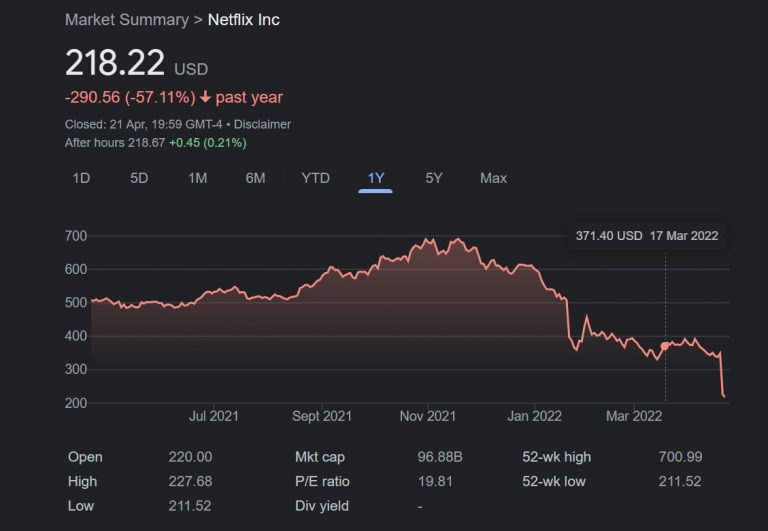A detailed screenshot of Netflix Inc.'s stock performance is displayed, featuring an informative stock chart. In the top left corner, the section is titled "Market Summary" in gray with a greater-than symbol leading to "Netflix Inc." in white text. Below, the current stock price is highlighted at $218.22 USD. Just beneath, the stock's performance over the past year is shown in red, indicating a significant decline of $290.56, or -57.11%, depicted with a downward arrow.

The status is marked as "Closed" with the precise date and time: April 21, 1959 GMT-4, along with a disclaimer. Subsequent to this status update, the after-hours price is shown in green at $218.67, reflecting a modest increase of $0.45, or +0.21%.

The chart itself provides a detailed visual representation, with the y-axis ranging from 200 to 700. The x-axis is labeled with various dates. At the top of the chart, there are filtering options to view the data over different periods: one day, five days, one month, six months, and so on. The meticulous layout aids in comprehensively understanding Netflix Inc.'s stock trends and performance over time.